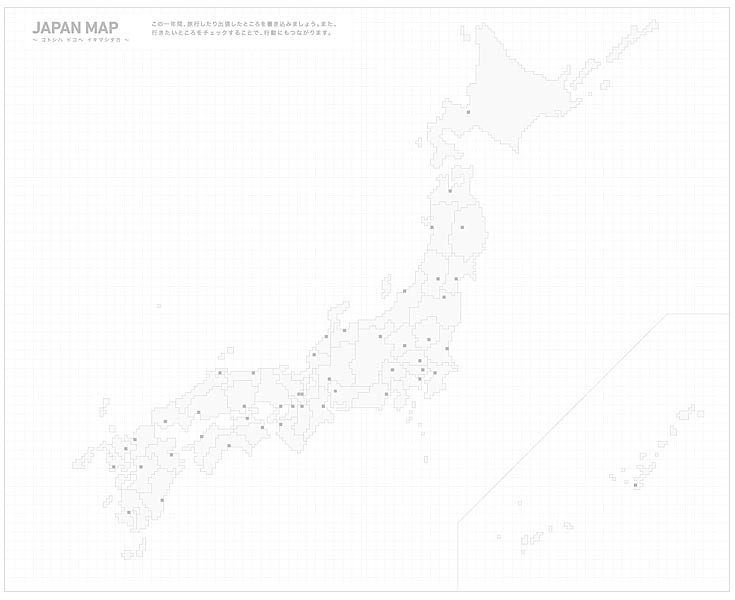The image is a low-contrast, pixelated map of Japan with the main islands and some smaller northern islands displayed. The top left corner features the label "Japan Map" in medium gray, accompanied by Japanese text below and to the right in two lines. The map itself is rendered on a very light gray dotted grid background, making it difficult to discern details. The islands of Japan are outlined in an extremely pale green or off-white hue, with dark dots signifying major cities or capitals. However, no city names or additional markings are visible, making the map appear somewhat vague and unclear. An inset in the bottom right corner displays smaller northern islands, completing the map's depiction.